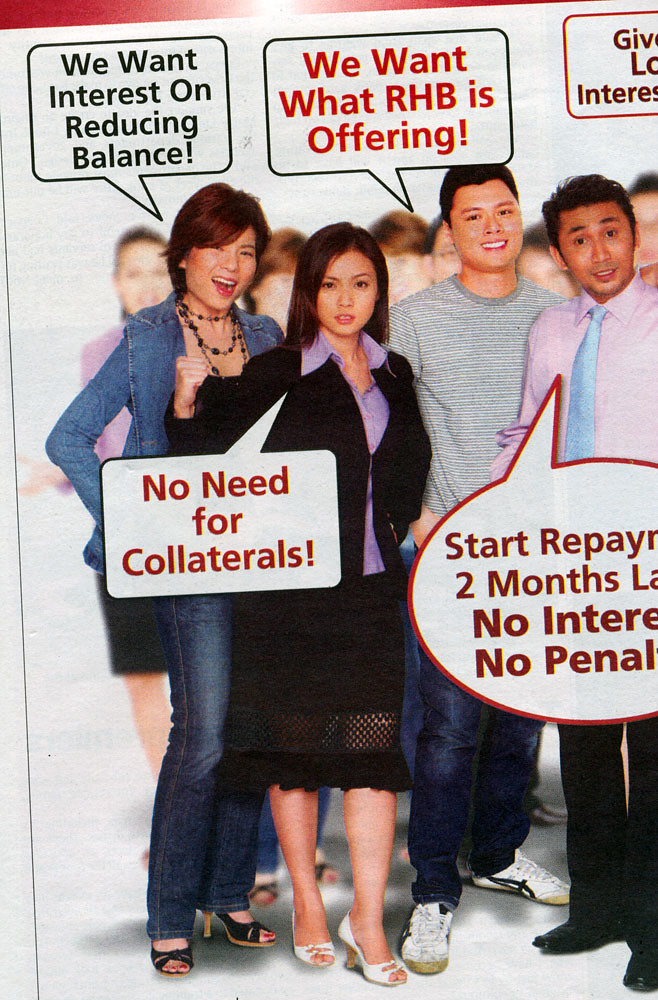The promotional image features a crowd with a focus on four individuals in the front, each accompanied by a speech bubble conveying different messages about banking products. On the far left, a woman dressed in a blue jean business suit, black and brown high heels, and a necklace has a speech bubble that reads, "We want interest on reducing balance" in black text. Standing to her right, another woman is wearing a black skirt, black coat, and a purple button-up shirt, with a red-text speech bubble stating, "No need for collaterals." Next to her, a man in blue jeans and a white and gray striped short-sleeved shirt has a speech bubble above him saying, "We want what RHB is offering" in red text. The final visible individual, a man dressed similarly in casual attire, has a partially cut-off speech bubble that reads, "Start repaying two months later. No interest, no penalties." The scene gives the impression of a dynamic, slightly distorted photograph, possibly altered for emphasis, set against a background of blurred faces, creating a sense of urgency and appeal for the banking services advertised by RHB.